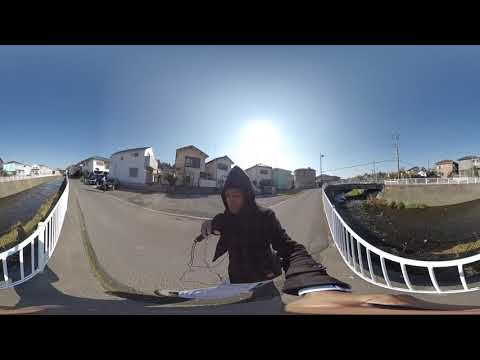The image portrays an outdoor scene of a man taking a selfie in front of a clear blue sky on a sunny day. The photo is notably distorted, likely due to a wide-angle lens, causing the resolution to appear stretched and curved. The man is centrally positioned in the image, wearing a black hoodie with the hood up, and a pair of white shoes. While his face isn't fully visible, his light skin can be discerned. His hand is prominently held up to the camera, making it appear unusually large due to the angle; he's possibly holding something that resembles a jump rope or wires. The background features a typical neighborhood setting with houses lining both sides, separated by white fences. The scene also includes two water-filled canals or ditches, fenced off for safety, giving the impression of an elevated area, possibly a bridge. The houses in the background vary in height, some being taller condo-like structures. The overall setting is well-lit under the bright sun with a completely cloudless sky.